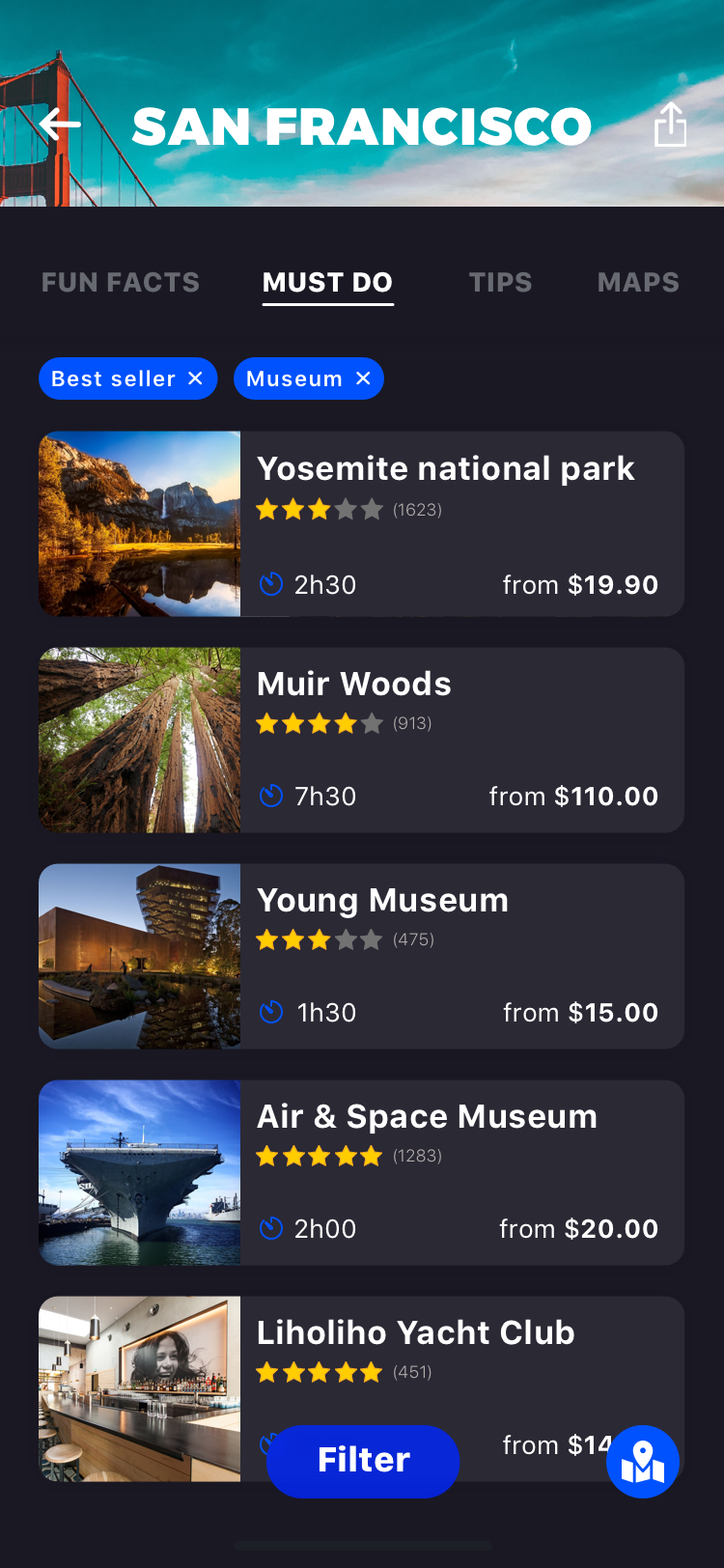**San Francisco Attractions Overview**

At the top of the image, the title "San Francisco" appears against a backdrop of the sky, with a slight glimpse of the iconic Golden Gate Bridge. Below the title, there are boxes labeled "Fun Facts," "Must-Do," "Tips," and "Maps," providing useful information for tourists.

Blue selection filter boxes labeled "Best Seller" and "Museum" help refine the choices of attractions. A list of various attractions follows, each accompanied by a brief description, rating, duration, and starting price, along with representative pictures:

1. **Yosemite National Park**: Rated three stars, this attraction is two hours and 30 minutes away and costs from $1,990. The picture shows a scenic water cave.
  
2. **Muir Woods**: With a four-star rating, this destination is seven hours and 30 minutes away and prices start at $110. The image depicts serene, towering trees.
  
3. **de Young Museum**: This three-star museum is an hour and 30 minutes away, with entry fees starting at $15. The photo features a large building with a distinctive, inverted pyramid structure on a concrete slab.
  
4. **Air and Space Museum**: Boasting a five-star rating, this museum is two hours away with tickets starting from $20. The visual shows a ship.
  
5. **Lino Hilo Yacht Club**: Rated five stars, this club is 14 minutes away with prices starting at $5. The image shows an interior featuring a painting and a bar, partially covered by a small map with a pin logo.

Each listing provides key information and a visual preview to help visitors select their desired activity or destination in and around San Francisco.